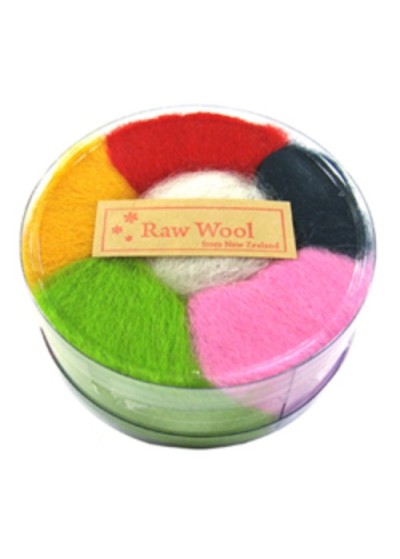The image depicts a transparent, circular plastic container neatly filled with six different-colored bundles of woolen yarn. The colors, arranged in a clockwise manner, are red, black, pink, green, yellow, and white, with the white yarn positioned centrally in the container. A tag on the lid prominently reads "raw wool," with additional, less legible text mentioning New Zealand. The container sits against a stark white background, suggesting a studio setting typically used for product photographs.